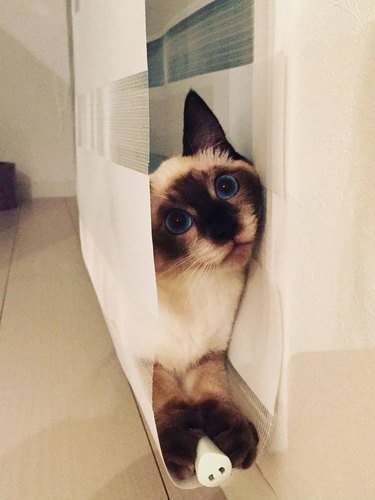In this image, there is a Siamese-style cat characterized by cream and tan fur with distinct dark brown and black markings. The cat has striking blue eyes and is seated between white blinds that are pulled down. Its dark brown or black nose features a brown marking that runs up between its eyes, stopping at its forehead. The curious-looking cat, with its head tilted against the wall, is resting its paws on a white pole. The room has off-white, cream-colored walls and tiles on the floor. Visible behind the cat is a white curtain with a subtle greenish or blue pattern. The cat's relaxed pose amidst this bright environment brings a gentle and inquisitive ambiance to the scene.